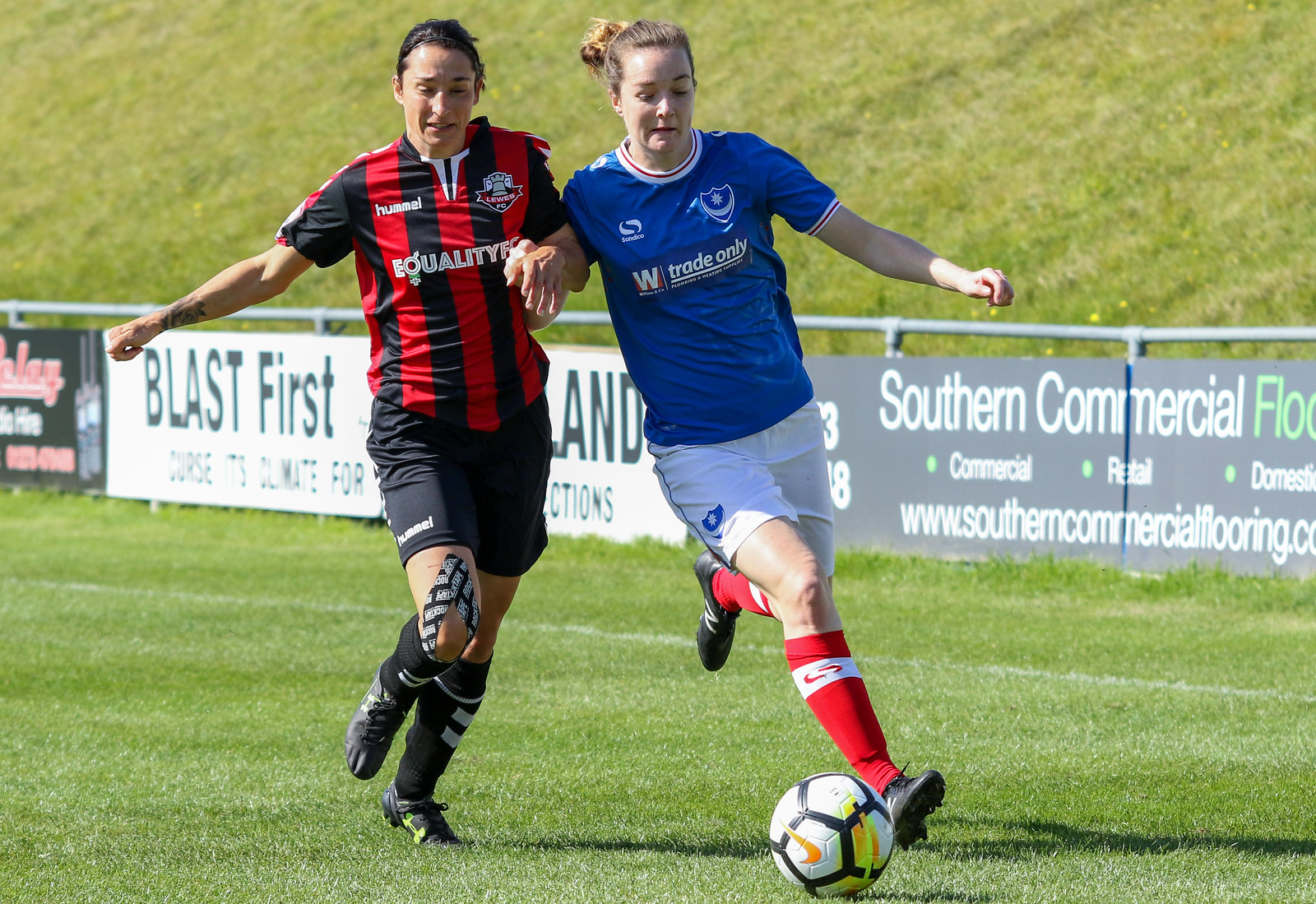In an action-packed outdoor soccer match on a lush green field bordered by a sloping grassy hillside, two female players are intensely vying for control of the ball. The scene is marked by a series of advertisement banners along a fence separating the pitch from the hill, one of which reads "Southern Commercial Flooring," and another that says "Blast First." These banners form the backdrop to the spirited contest between the players. On the left, a brunette with her hair tied up is dressed in a red and black vertically striped jersey, black shorts, black socks, and black cleats. She wears a black and white knee bandage on her right knee. Her opponent on the right, with lighter hair also tied up, sports a blue jersey with the words "Trade Only" across the front, white shorts, red socks, and black cleats. Both players are fixated on the predominantly white soccer ball marked with yellow and blue stripes, their bodies almost pushing against each other in a fierce struggle for possession. The detailed scene captures the dynamic energy and competitive spirit of the match.